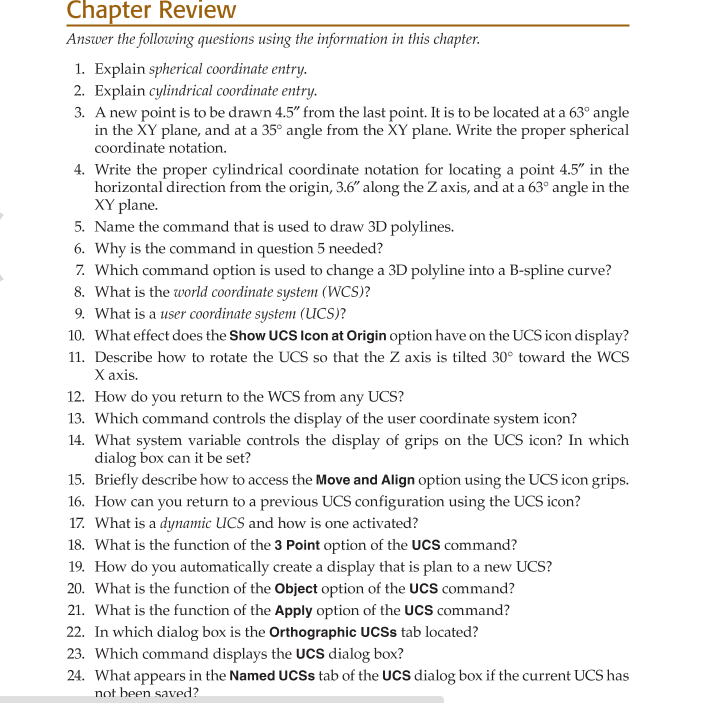This image depicts a textbook's chapter review page, specifically for a math or programming subject. At the top of the page, "Chapter Review" is prominently displayed in an orange font. A long divider line, matching the brownish-orange color of the title, separates the header from the content below. Directly beneath this, italicized text instructs students to "answer the following questions using the information in this chapter." 

The main content consists of a list of 24 review questions, each numbered consecutively from 1 to 24. The questions are printed in black text on a crisp white background, with each question carefully spaced. Some examples of questions include:

1. Explain spherical coordinate entry.
2. Explain cylindrical coordinate entry.
3. A new point is to be drawn 4.5 inches from the last point. It is to be located at a 63-degree angle in the XY plane and at a 35-degree angle from the XY plane. 

At the very bottom of the page, there is a faint light gray line, subtly marking the end of the content area. The overall layout is clean and well-organized, allowing the reader to easily focus on the questions presented.